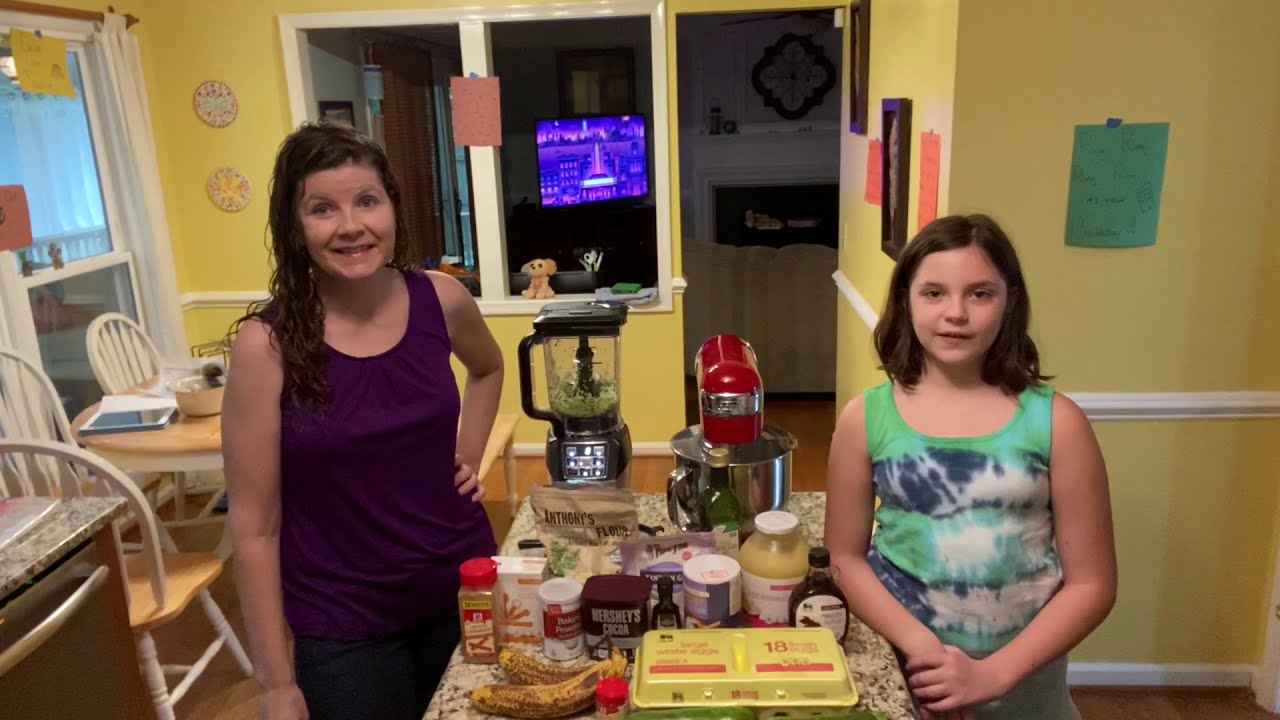In this indoor kitchen scene, an older woman and a young girl stand on either side of a central countertop island laden with various cooking ingredients and utensils. The older woman, positioned to the left of the island, has shoulder-length wavy brown hair, wears a purple sleeveless blouse, and dark jeans. She stands with a hand on her hip, smiling. The young girl, on the right side of the island, has short brown hair and dons a green, blue, and white tie-dye tank top. Her left arm rests on the island, which holds items such as ripe bananas, a carton of eggs, a jar of applesauce, Hershey's cocoa, and various spices and flour. Additionally, a steel mixing bowl with a red top and a black and silver blender with green highlights are present.

The room is warmly decorated with yellow wallpaper. Behind the older woman is a light wood table with white-accented chairs, and some items, which might include books and a bowl, are placed on the table. A window with a white curtain sits to the far left, and paintings and handwritten sheets adorn the walls. There is also a doorway in the background, opening into what looks like another room, possibly a family room with a television that is currently on. The scene seems like a moment from a cooking video, capturing a warm and engaging kitchen activity.